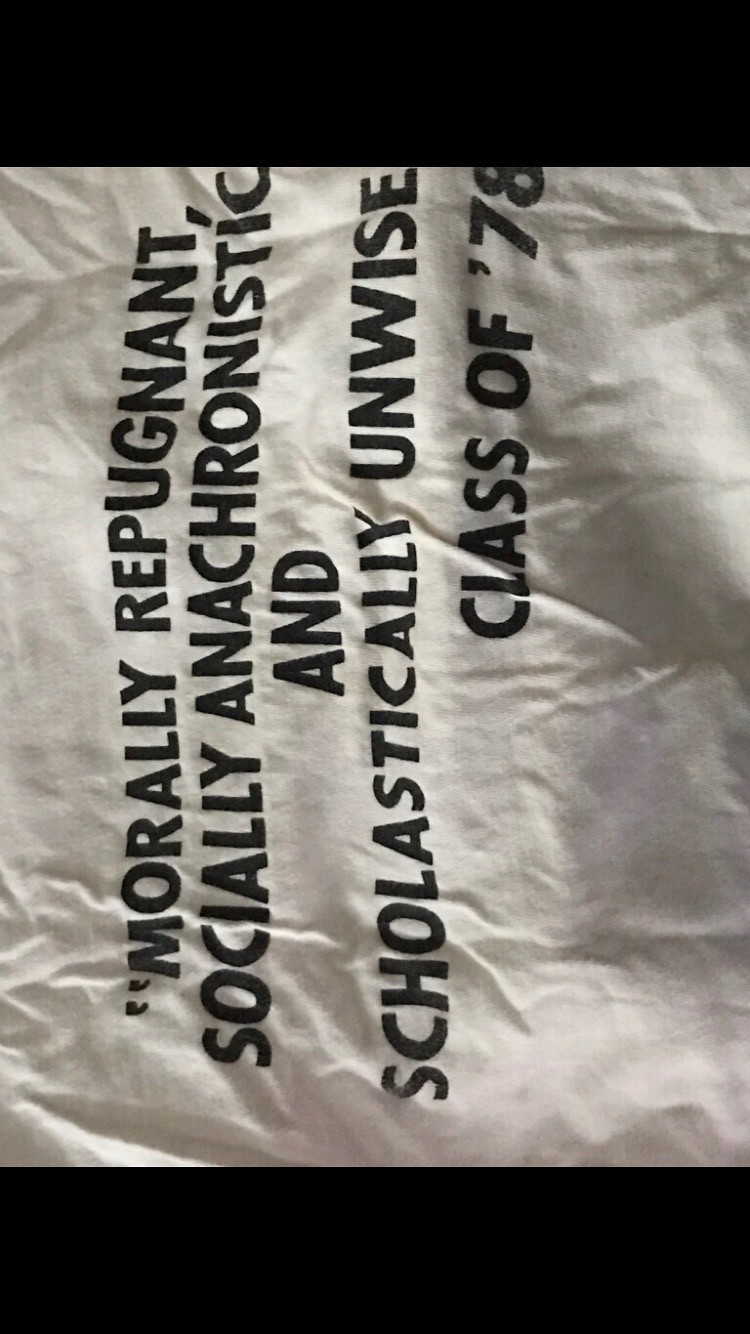This vertical photograph features a wrinkled white cloth boldly printed with the following text in all capital, black letters: "MORALLY REPUGNANT, SOCIALLY ANACHRONISTIC AND SCHOLASTICALLY UNWISE, CLASS OF '78". The stark lettering stands out prominently against the plain background, creating a sharp contrast. Thick black bars frame the top and bottom of the image, further emphasizing the central text. There are no living beings, plants, buildings, signs, or vehicles present, making the banner the sole focal point of this color photograph.